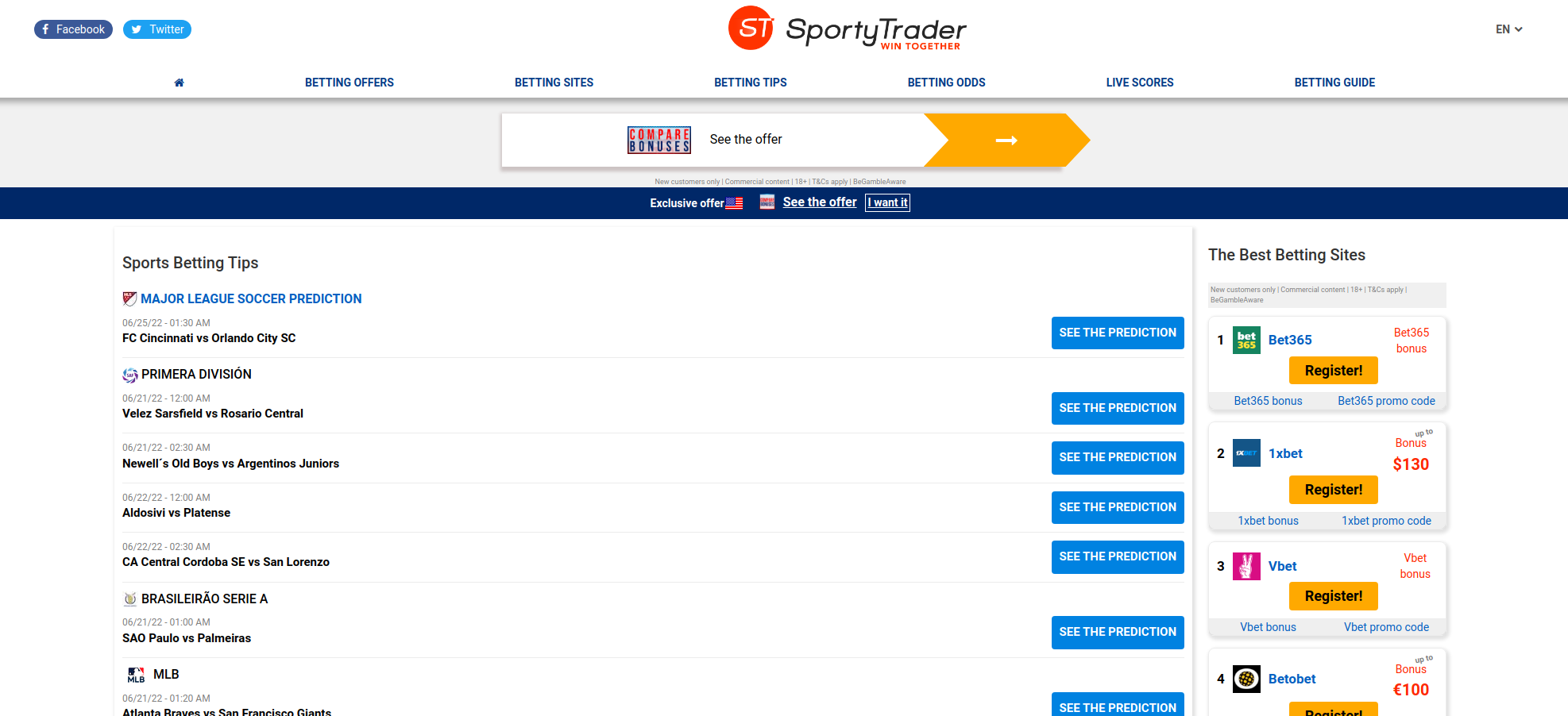The website, Sporty Trader - Win Together, features a clean and informative homepage with several key elements. In the upper left corner, there are icons for Facebook and Twitter. A white strip spans the top of the page, with "Sporty Trader" prominently positioned in the center. On the upper right, there's a language selection drop-down menu marked with "EN."

Below the white strip, a menu offers links to "Betting Offers," "Betting Sites," "Betting Tips," "Betting Odds," "Live Scores," and the "Betting Guide." In this section, there is also a prompt to "Compare Bonuses" and "See the Offers," housed in a white rectangle that tapers to a point on the right side. Adjacent to this, the rectangle transitions from white to orange and features a white arrow and the disclaimers: "New customers only, commercial content, 18+, T&Cs apply, be gamble aware."

A blue bar below this section highlights an "Exclusive Offer" accompanied by an American flag and a button labeled "See the Offer" and "I want it."

Further down on the left side, the site lists "Sports Betting Tips" with upcoming games such as "Major League Soccer Predictions" for June 25, 2022, at 1:30 a.m., featuring FC Cincinnati versus Orlando City SC. Another entry previews the "Primaria Division" match on June 21, 2022, at 12 a.m., between Vélez Sarsfield and Rosario Central.